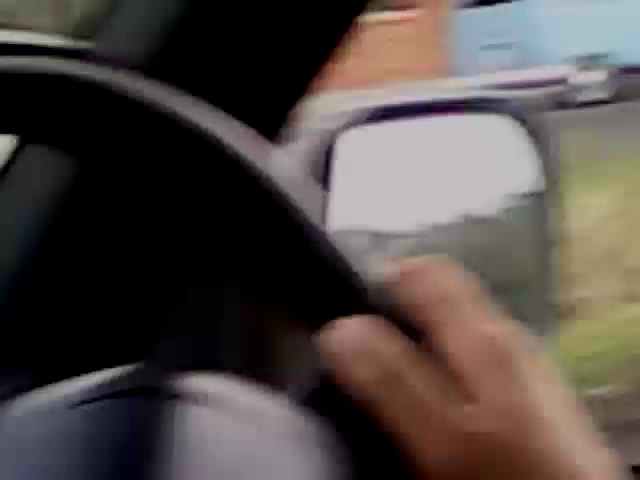The image is an extremely blurry and pixelated photograph taken from inside a car with the steering wheel positioned on the right side, suggesting it is not in America. The focus of the image is on a black or dark gray steering wheel with a medium skin-toned hand gripping its side, notably showing the thumb and part of the forefinger. The background visible through the windows includes a green expanse of grass and various indistinct buildings or structures; one appears to be light orange while another beside it is light blue. There may also be a vehicle adjacent to the blue structure. The side window and portion of the door frame are visible, with reflections indicating a possibly grassy landscape outside. Despite an attempt to observe details, the image's overall quality remains significantly degraded and pixelated.